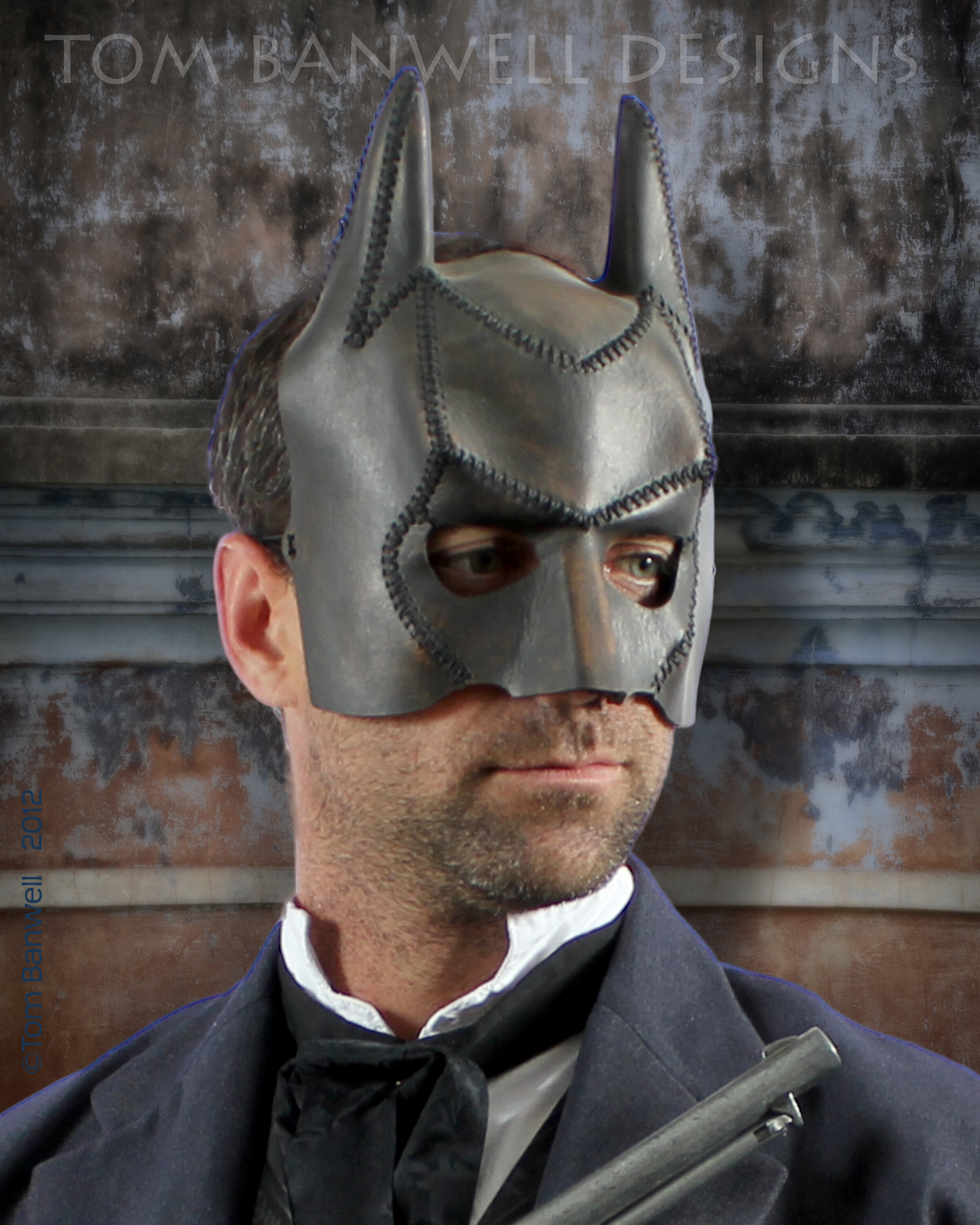This image captures a striking portrait of a man dressed in an elaborate, vintage ensemble. The top of the photograph features semi-transparent white text that reads "Tom Banwell Designs." Dominating the frame is a close-up of a man wearing a Victorian-era, leather Batman-style mask adorned with stitching and characteristic bat ears. The mask covers the top of his head down to his nose, with cutouts for his eyes. His facial features include dark brown hair tinged with gray and a five o'clock shadow.

He sports an old-fashioned tuxedo with a white collared dress shirt and a loosely tied black bow tie, complemented by a black dress jacket. Held in his right hand is an old, rusted silver gun, with part of the barrel visible, pointing upward to the right of the frame. The background reveals an aged, distressed wall with a patina and faded layers of browns, blues, and orange, suggesting the photograph was taken in an abandoned or old house. The overall composition blends elements of vintage fashion and a rugged, antiquated setting, creating a visually evocative scene.